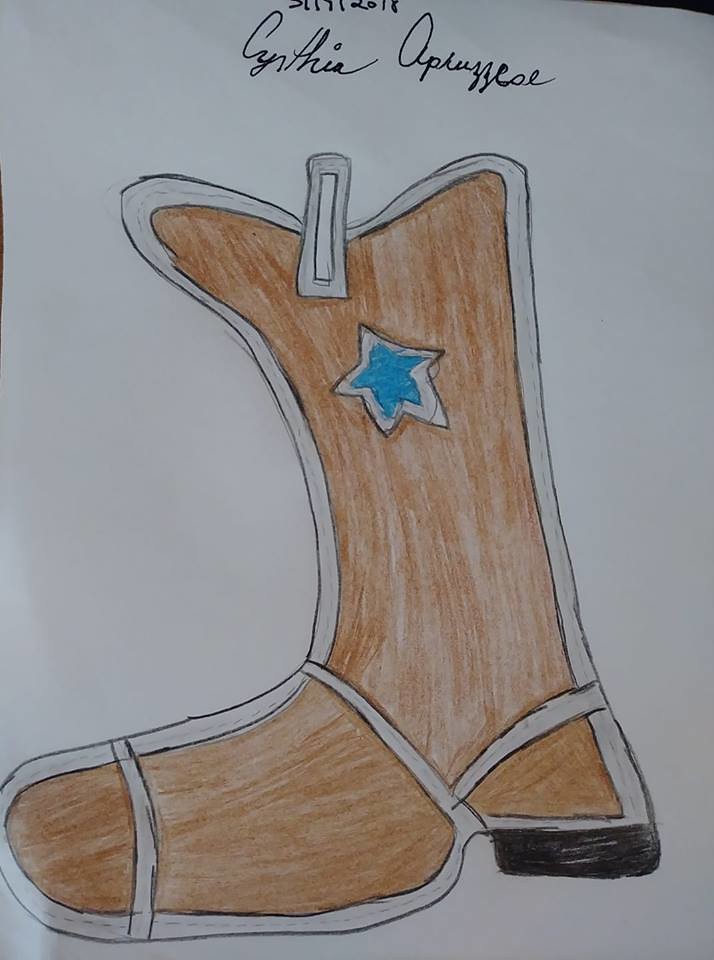This image features a child-like drawing of a cowboy boot on a plain white piece of paper, created using colored pencils. Across the top of the paper, there's a date, "03/17/2017," followed by the artist's name, "Cynthia," written in black ink, though the last name is illegible, appearing as a loose and scraggly cursive. Dominating the center of the image is the cowboy boot drawn in a flat, two-dimensional style. The boot is light brown, outlined in white, with a prominent blue star in the upper middle, also bordered in white. Distinctive features include a black heel and large white lines that run across the toe, back, and heel of the boot. Additionally, there's a gray clip or tag at the top, contributing to the boot's rudimentary yet charming aesthetic.